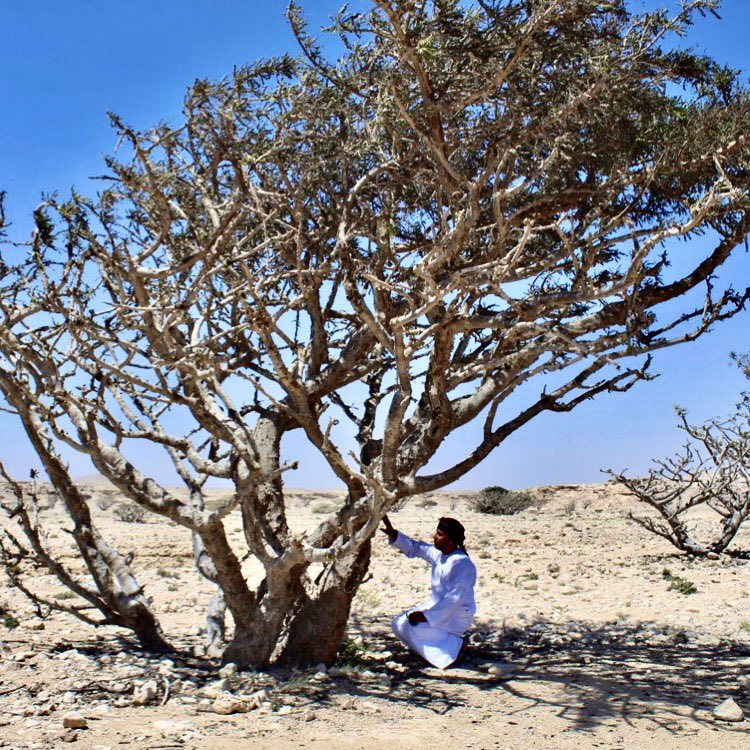In the middle of a vast and arid desert landscape, a striking scene unfolds on an exceptionally sunny day. The backdrop showcases a clear, cloudless blue sky, intensifying the bright, hot atmosphere. Dominating the foreground is an ancient, gnarled tree with numerous barren branches and sparse green foliage concentrated at the top. The tree stands firmly in the dry, sandy ground, with a few scattered rocks and small dead bushes dotting the terrain.

Kneeling at the base of the tree is a young man dressed in a long, white, long-sleeved robe that resembles a toga. His attire is complemented by a dark headscarf wrapped around his head. The man appears to be deeply engaged with the tree, his outstretched hand tenderly touching its weathered bark. The sun casts a sharp shadow directly below the tree and the crouching figure, emphasizing the midday heat and starkness of the environment.

To the right of the man, another smaller, nearly leafless tree stands, adding to the scene's desolate beauty. The overall composition of the image evokes a sense of solitude and reverence in this harsh yet captivating desert setting.